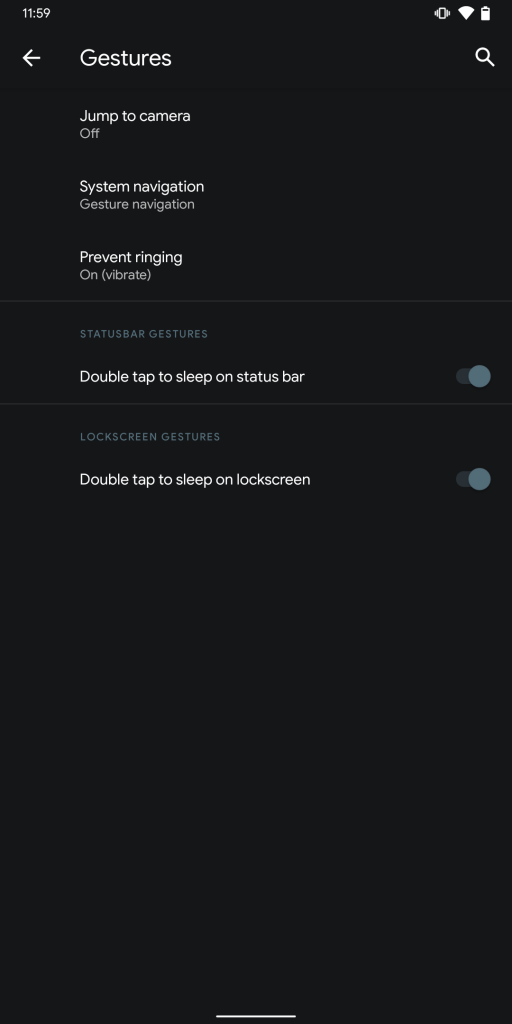This screenshot, likely taken on a smartphone, measures approximately 3.5 inches by 5 inches. At the top left corner, it displays the time as 11:59. The top right corner features several icons: a possible vibrate symbol, Wi-Fi connection status, and an almost full battery indicator. 

The screen background is black, contrasting sharply with the thin white text. Just below the status bar, the word "Gestures" is displayed, accompanied by a left-facing arrow. To the right of this word, there is a search icon. 

Scrolling below this header, several settings are outlined in small white print. The first setting reads "Jump to camera: Off." Further down, under the "System navigation" section, "Gesture navigation" is noted. Following this, the "Prevent ringing" feature is listed as "On" with the mode set to "Vibrate."

The next segment, labeled "Status bar gestures," specifies that "Double-tap to sleep on status bar" is active, with a toggle switch available for enabling or disabling this feature. Lastly, in the "Lock screen gestures" section, "Double-tap to sleep on lock screen" is also enabled, with a similar sliding switch for toggling the setting on or off.